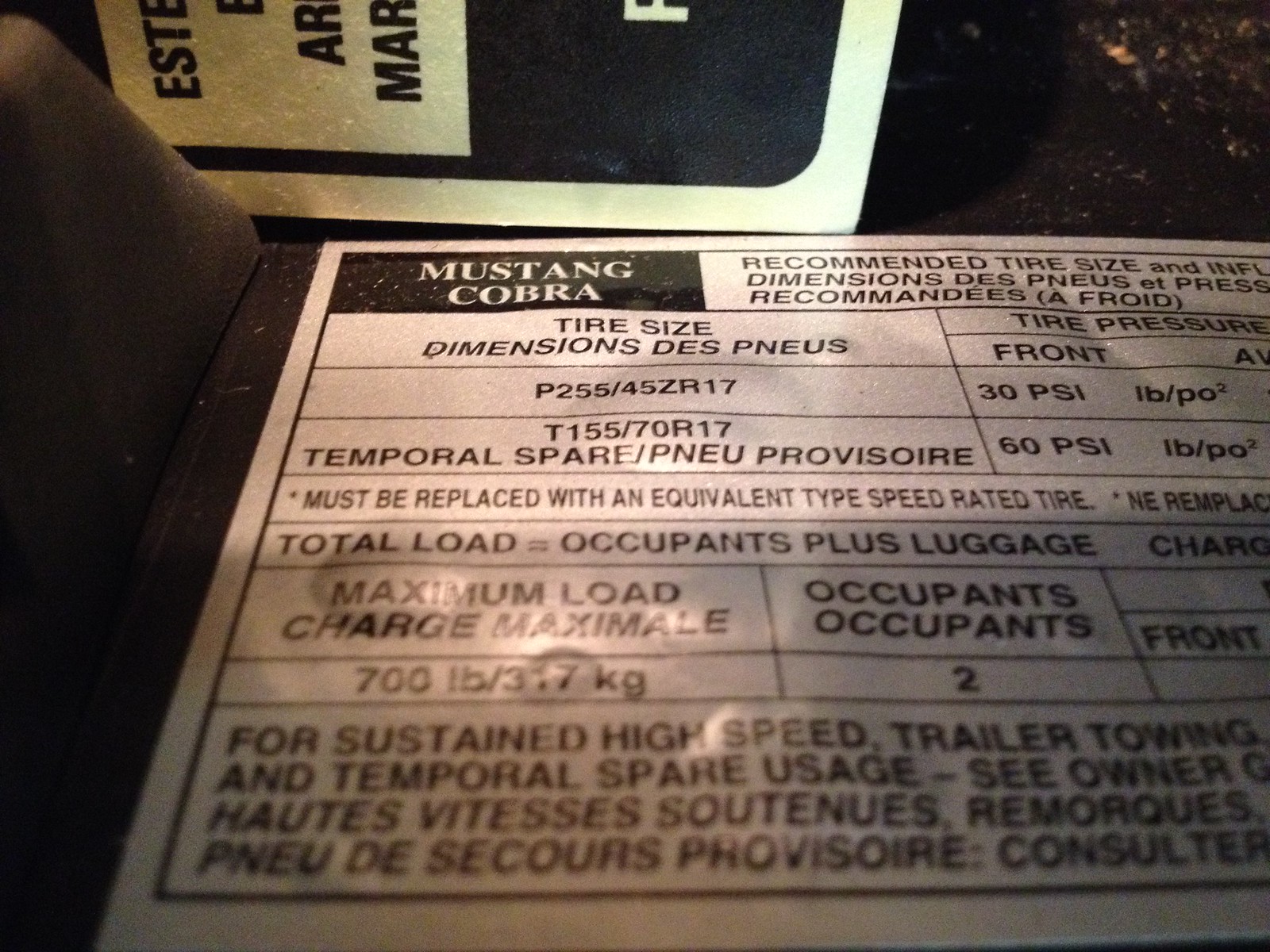This is a detailed photograph of a white sign with black text located inside the door well of a Mustang Cobra, giving specifics about tire specifications and vehicle load capacities. The sign is somewhat cropped, focusing on essential information. It clearly states "Mustang Cobra" at the top left. The recommended tire size is listed as P255/45ZR17, with a front tire pressure of 30 PSI and a temporal spare tire size of T155/70R17, which should be inflated to 60 PSI. The sign further emphasizes that the temporal spare must be replaced with an equivalent speed-rated tire. For a two-seater Mustang, the maximum load capacity, combining occupants and luggage, is 700 pounds (317 kilograms). The instructions also reference high-speed trailer towing and advise consulting the owner's manual for more details. In the background, part of the car's interior is visible, providing context to the information presented on the sign.